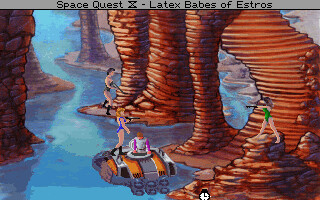This image is a screenshot from an older video game, likely from the 80s or 90s, titled *Space Quest*. The top of the image features a gray banner with the game's title in black print along with a dash that introduces the subtitle "Latex Babes of Estros." 

The scene depicted appears to be an elaborate cave with blue water flowing through it. Surrounding the water are large columns made of stone and brick that resemble traditional cave formations. There is a small, somewhat futuristic-looking boat or machine floating on the water, and a stopwatch or alarm clock displayed at the bottom center of the screen.

Several cartoonish characters are present in the image, including multiple young women wearing one-piece swimsuits in various colors such as green and black. These characters also hold guns. Another notable figure is a man, possibly inside a tank or another machine, observing the scene. The overall aesthetic and characters suggest a stylized, somewhat humorous approach typical of vintage video games.